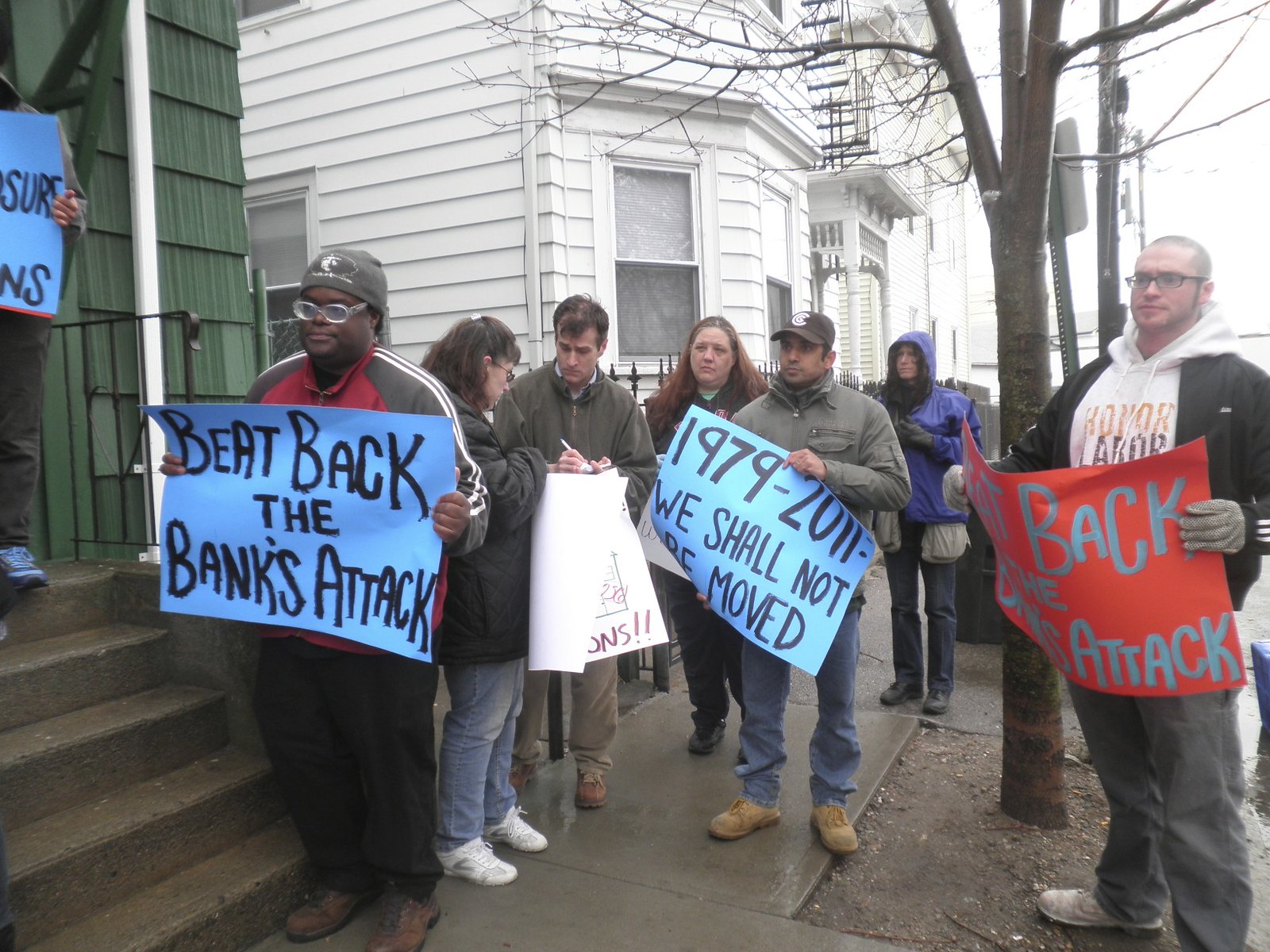The image depicts a protest happening in a residential neighborhood on a cloudy, rainy day. The protesters are gathered on a wet sidewalk at the base of concrete steps leading to a green shingled house, with an older white shingled house also visible in the background. There is a tree along the street, adding to the residential setting. The crowd is composed of people dressed in cold weather attire, suggesting it is a chilly day.

At the center of the image, a group of protesters is holding up handmade signs on construction paper. The signs display messages like "Beat back the banks’ attack" and "1979 to 2011, we shall not be moved." One prominent sign is held by a Black man wearing white-rimmed plastic glasses, a gray beanie, and black pants. A Hispanic man beside him holds a blue sign with the same slogan. Another protester, a white man in a black jacket and black-rimmed glasses, holds an orange sign with blue text, though the exact wording is not visible.

A diverse crowd of onlookers and additional protesters can be seen in the background, contributing to the sense of community involvement in this local demonstration against a bank's actions, possibly attempting to displace residents from their homes.